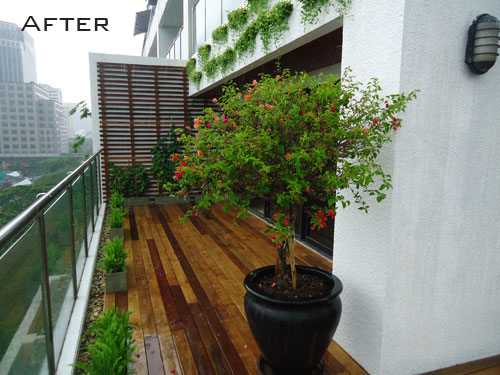This photo captures a sophisticated urban balcony or rooftop deck with teak or hardwood flooring, featuring a blend of dark and light planks, glistening with recent rain. The balcony, part of a white stuccoed concrete building, is enclosed by a transparent glass and metal safety rail, showcasing an expansive view of the city’s high-rise office buildings. A bush with small red flowers, potentially a trained rose or fuchsia, sits in a black pot beside a green-laden trellis on the far end, while several rectangular pots containing ferns line the edge of the deck alongside decorative pebbles. Additional greenery cascades from above, contributing to the lush ambiance of this elegant outdoor space. The sky is overcast, adding a gloomy yet serene atmosphere, and the word "AFTER" is inscribed in the upper left corner of the image, suggesting a transformation or renovation.